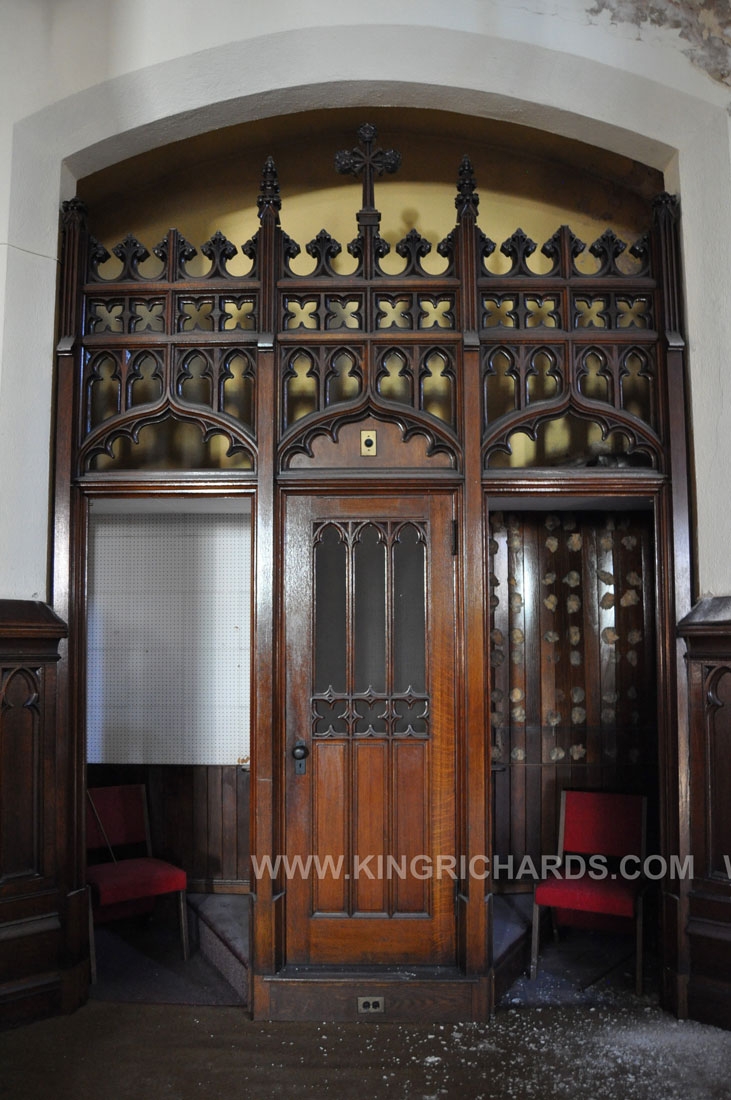This photograph captures the interior of an old church's confession booth, characteristic of a mid-20th century design. The booth features three doors—one in the center, presumably for the priest, which remains closed, and two side doors that are open, each revealing a red chair for the parishioners. The structure is crafted from beautifully stained brown wood, adorned with intricate scrollwork and a central cross. The booth stands atop a slightly elevated step, contrasting with the older wood floor of the church. The background includes an archway with a gradient from gray to white tiles. The rich color palette features mahogany, red, black, pale yellow, and brown hues. The craftsmanship and style suggest a Roman Catholic church.